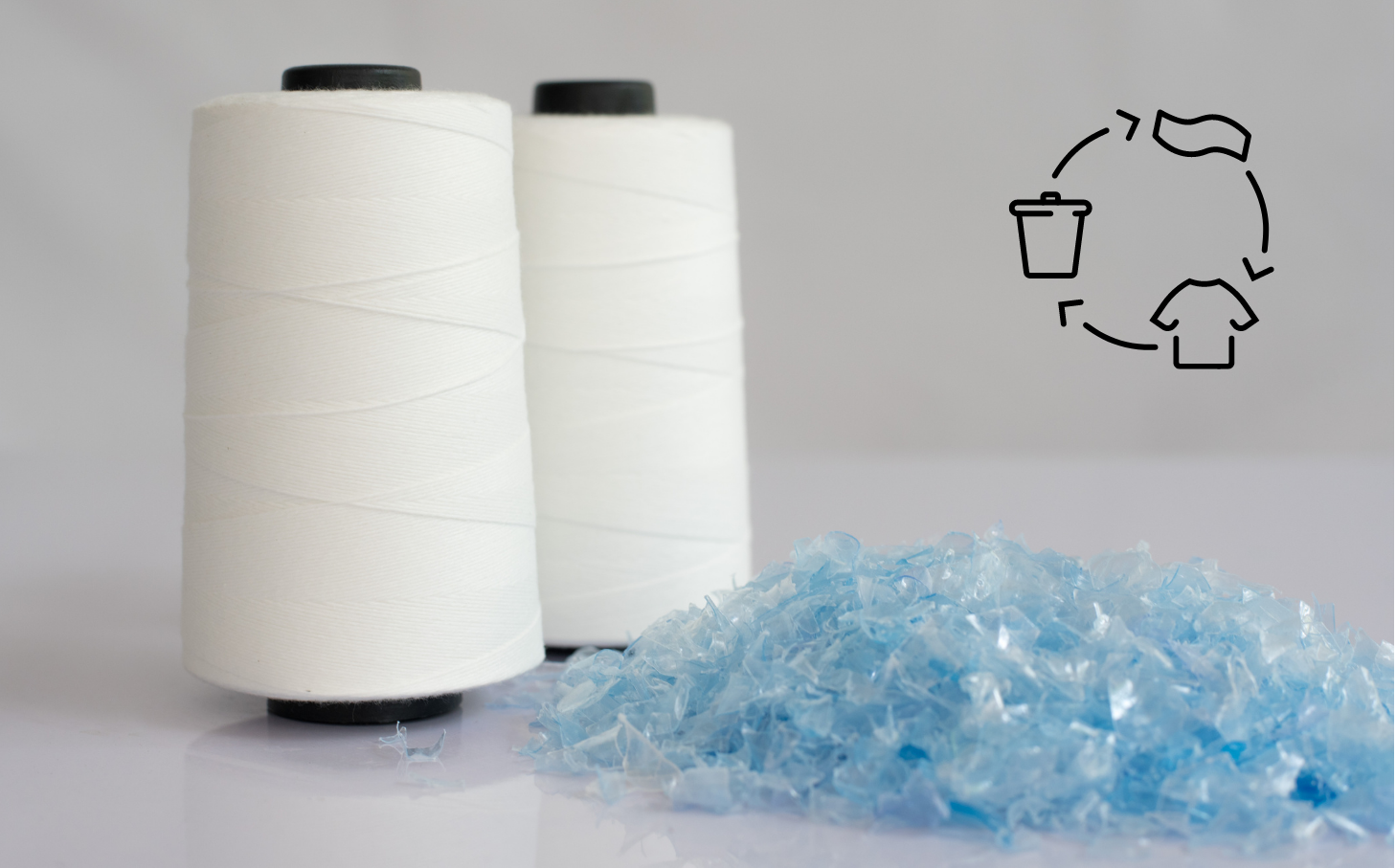The photograph, taken indoors, features a rectangular frame about five inches wide and three to four inches high. The background is split into two shades: the bottom half is light gray, seamlessly blending into the darker gray top half. In the upper right-hand corner of the image, there is a black graphic depicting a recycling process. This graphic includes three arrows forming a circle, with each arrow connecting different images: a garbage can on the left, a piece of cloth in the upper right, and a T-shirt in the lower right, illustrating the recycling cycle from disposal to fabric transformation.

On the lower right-hand side of the image, there is a pile of light blue plastic shards scattered on a shiny white surface. To the left of the plastic shards are two large spools of white twine or thread. These spools are mounted on black, cone-shaped cores that are narrower at the top and wider at the bottom. The minimalist recycling graphic suggests that the plastic shards might be part of a process where recycled materials are transformed into new products, such as the spools of twine displayed.